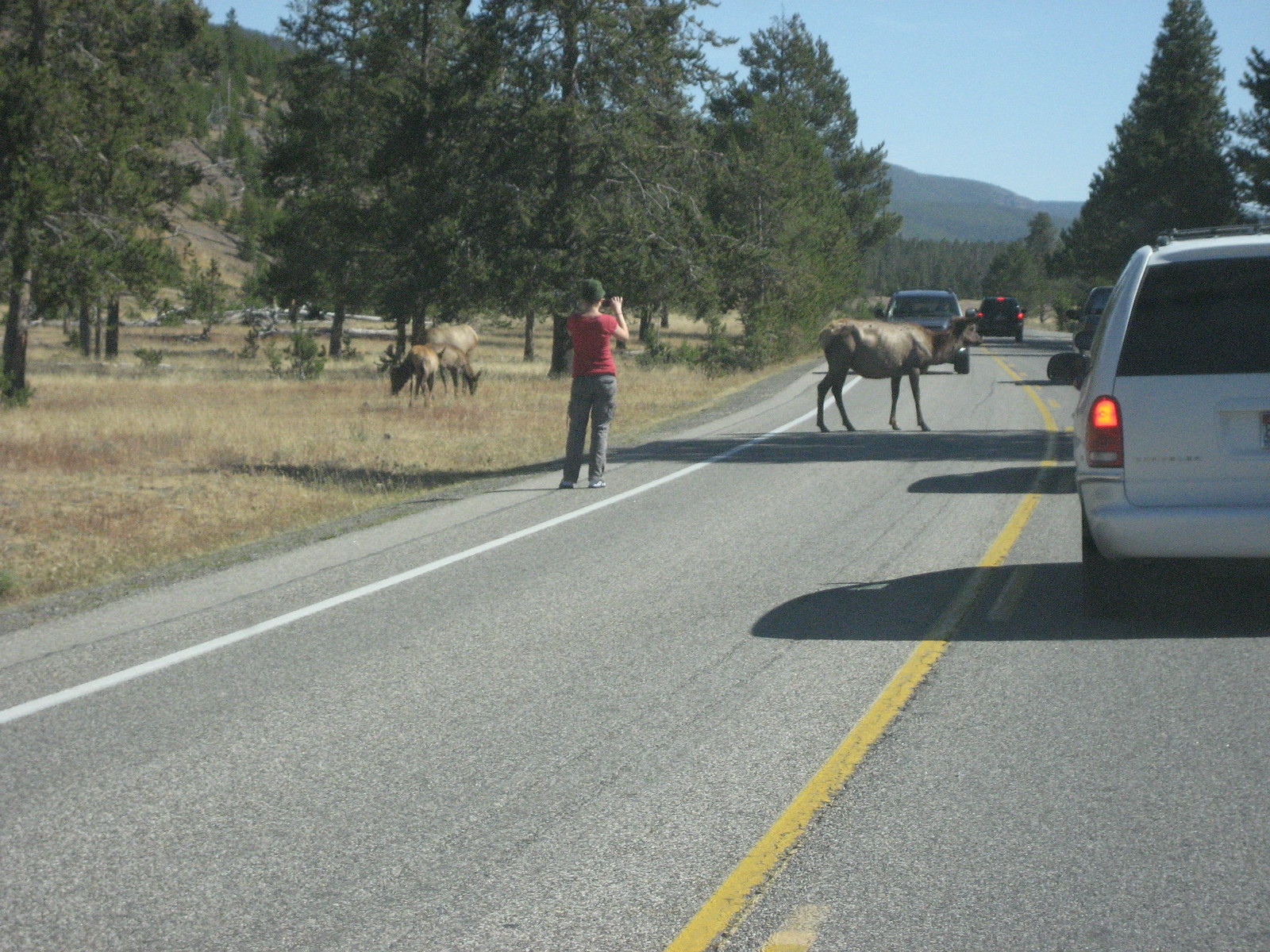A person in a red shirt and blue jeans stands on the road, capturing a photo. On the right side, a car with illuminated red taillights is driving forward, casting shadows to the left. Some animals are standing on the road, likely the reason the car appears to be moving cautiously. Behind the car, there is a drive-thru flanked by tall trees with lush, green leaves. The setting is a mountainous region with a hill to the left. In the far distance, the peak of a mountain is visible, blending seamlessly into the scenic landscape.